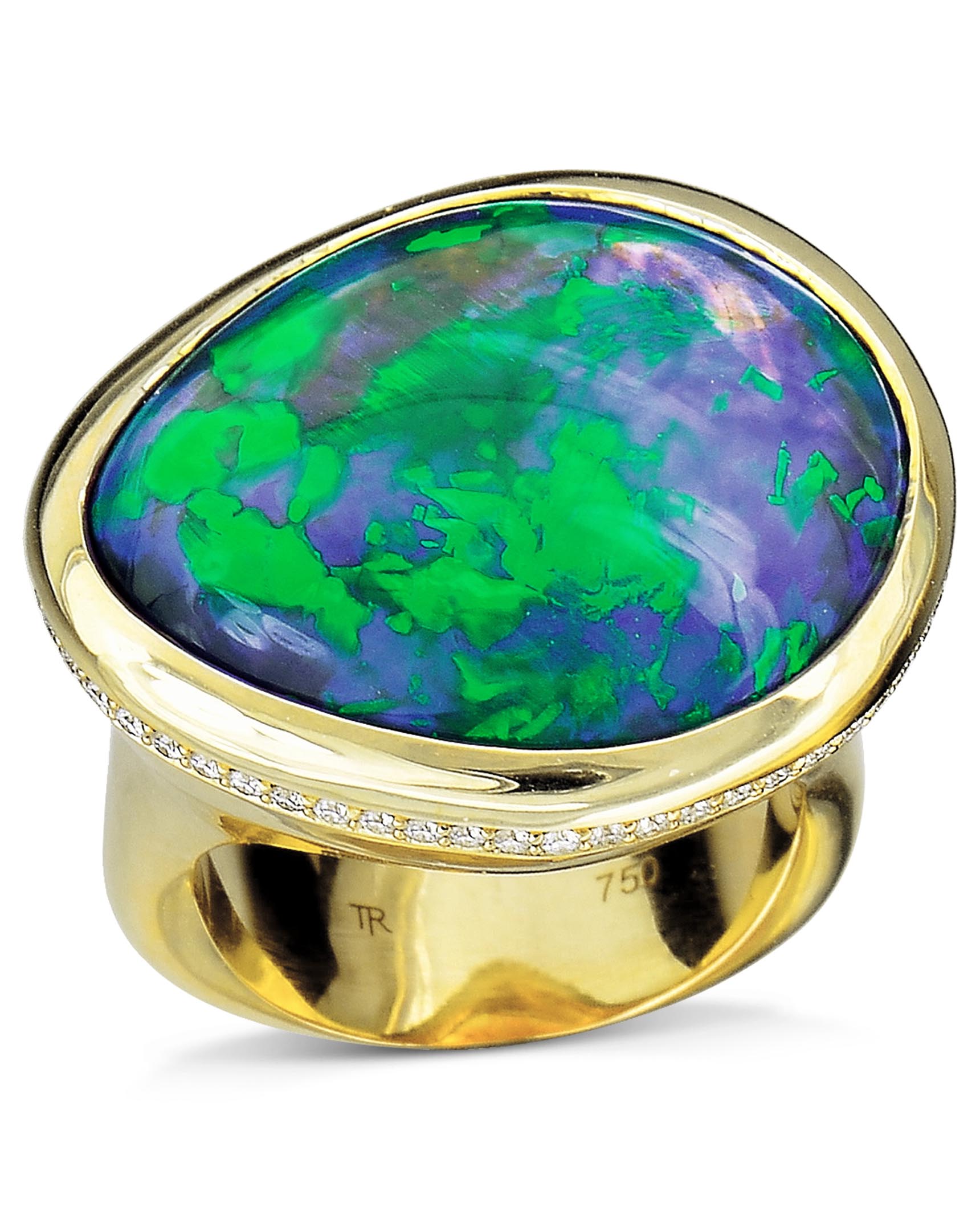In this well-lit close-up image set against a white background, a golden ring is prominently displayed. The ring, made from high-quality gold, features an intricate and captivating design. At the top sits a striking marbled stone, hues of blue and green blending in a pattern reminiscent of the Earth's surface. This central stone is encircled by a golden border, which is itself outlined by a ring of small, sparkling white diamonds, adding a touch of elegance and brilliance to the piece. On the inner band of the ring, the inscriptions "TR" and "750" are clearly engraved, indicating the maker's initials and the gold's purity. The image highlights every intricate detail of this exquisite piece of jewelry.